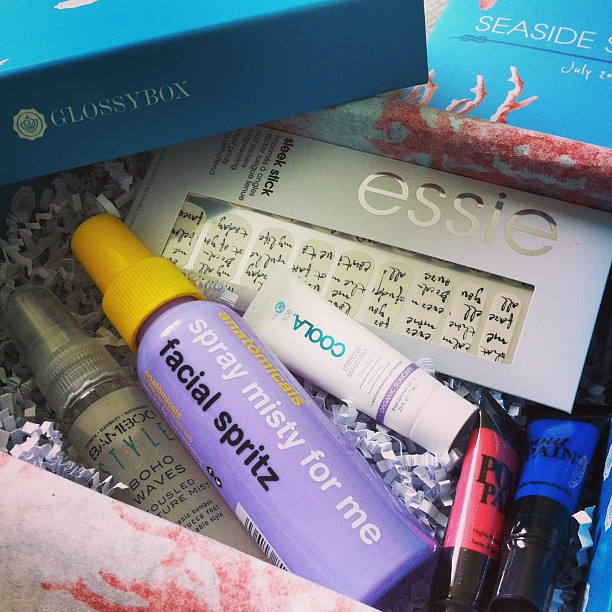This image shows the meticulously arranged contents of a Glossy Box gift box, designed for personal care and beauty. The lid, positioned in the top left-hand corner, is a sky blue color and prominently displays the "Glossy Box" logo in white. Atop the box, on the right-hand side, there's another sky blue paper featuring partial text that reads "Seaside July."

Inside the box, which features a visually appealing reddish tie-dye design, the items are nestled in crinkled white confetti packaging. Starting from the left, the first item is a tan bottle labeled "Bamboo-Style Boho Waves." Next to it is a purple bottle with a yellow cap that reads "Spray Misty for Me Facial Spritz" in a mix of black, white, and yellow fonts. Following this is a small white tube labeled "Kooler" or "Koola," suggesting skincare usage. Behind this tube is a larger gray box marked "Essie Sleek Stick," likely containing nail products or decorative stickers.

In the bottom right-hand corner, there are two small containers, one pink and one blue, possibly for eye shadow or another type of makeup. The assortment of bottles includes two regular-sized spray bottles and three smaller bottles, offering a variety of facial and body care products intended to pamper and rejuvenate.